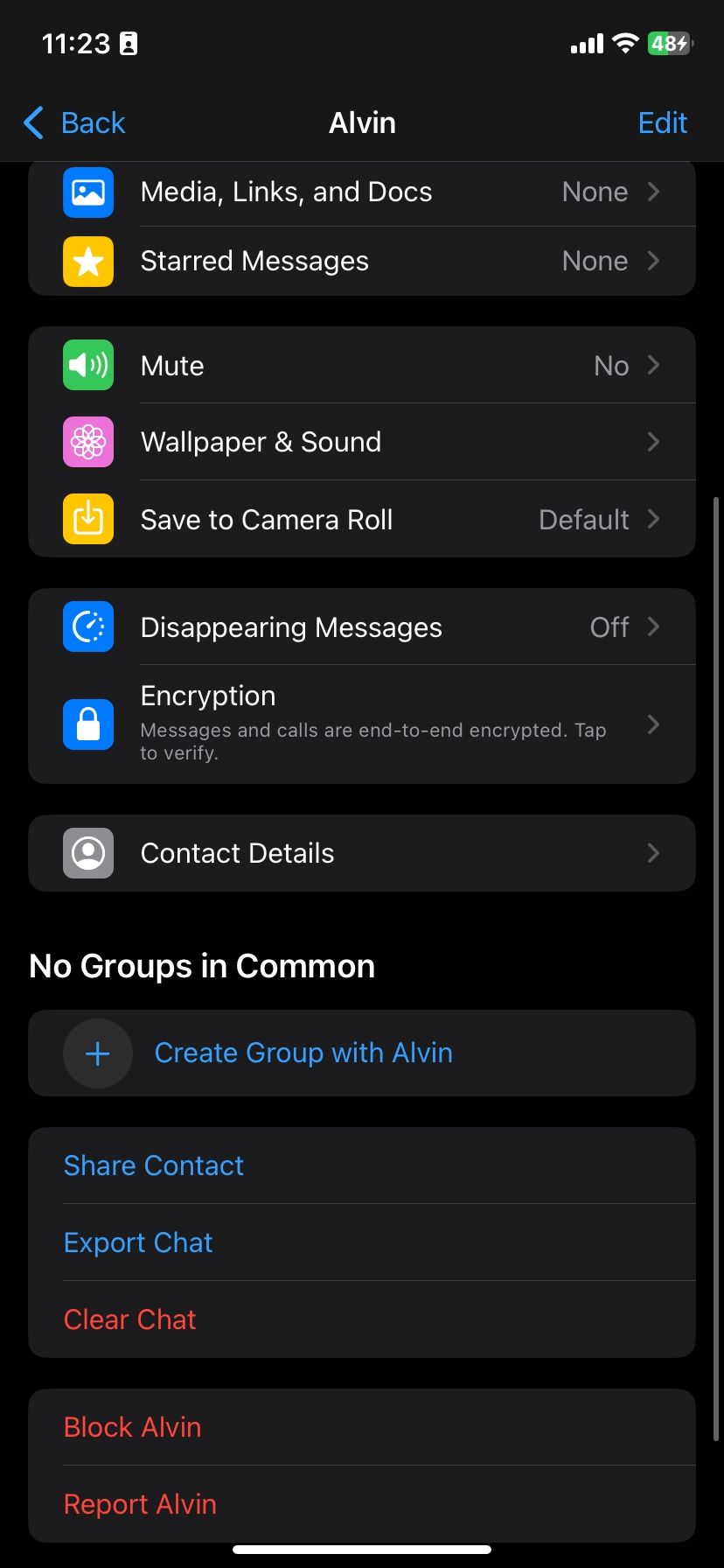The image depicts a phone screen showing a contact's detailed settings. At the top, the status bar displays the time "11:23" in white lettering, with signal bars and the Wi-Fi symbol to the right. Below this, the navigation bar features "Back" in blue lettering with a left-pointing arrow, the contact name "Alvin" in white lettering, and "Edit" in blue lettering to the right of the name.

The main section of the screen lists various settings and options, each with an icon to the left and a right-pointing arrow indicating further details can be accessed:

1. **Media, links, and docs** 
2. **Starred messages**
3. **Mute**
4. **Wallpaper & Sound**
5. **Saved Camera Roll**
6. **Disappearing messages**
7. **Encryption**
8. **Contact details**

Just below these options, there is a notification in white lettering that reads "No groups in common." Following this, there are additional options in blue lettering:

- **Create group with Alvin** (accompanied by a blue plus sign in a light black circle)
- **Share contact**
- **Export chat**

Towards the bottom of the screen, in red lettering, are options for:

- **Clear chat**
- **Block Alvin**
- **Report Alvin**